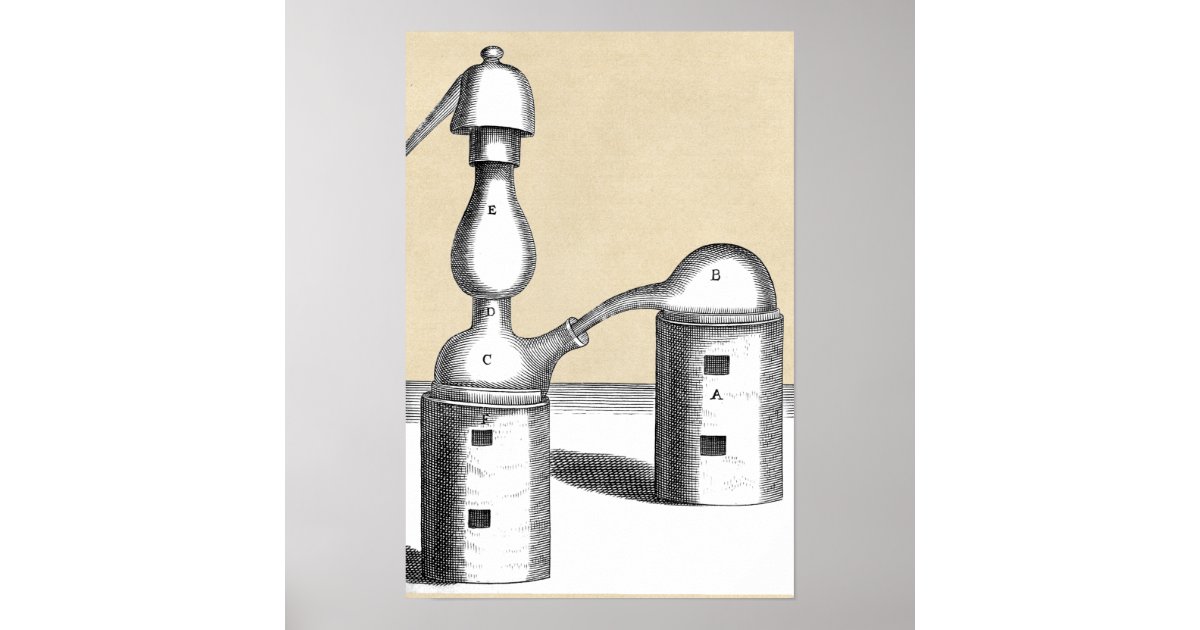The image depicts a black-and-white drawing of two cylindrical containers, resembling chemistry equipment or flasks, set against a square gray background with a beige rectangular picture or painting hanging vertically on it. Both cylinders have shading to give them depth, and they cast a shadow on the light-colored table they rest on. The cylinder on the right features a dark shadow behind it for further dimensionality.

The left container, which is labeled 'F' at the top, is topped with a small spherical funnel that narrows into a spout. Sitting atop the funnel is a bulbous structure marked 'E,' which is connected to an additional piece resembling a water faucet or pump. This container also has two small square windows punched into its surface.

The right container, labeled 'A,' has a similar structure. A round piece labeled 'B' fits into a smaller connector marked 'C,' and then into another labeled 'D.' This series of connections leads into a teardrop-shaped piece marked 'E,' which curves upwards into a smaller, upside-down pipe-like structure. From the bottom of this, another funnel extends and interlocks with the funnels on the adjacent container. The detailed shading and combination of three-dimensional drawing techniques, including a shadow on the table, contribute to the depth and realism of the objects depicted in the image.